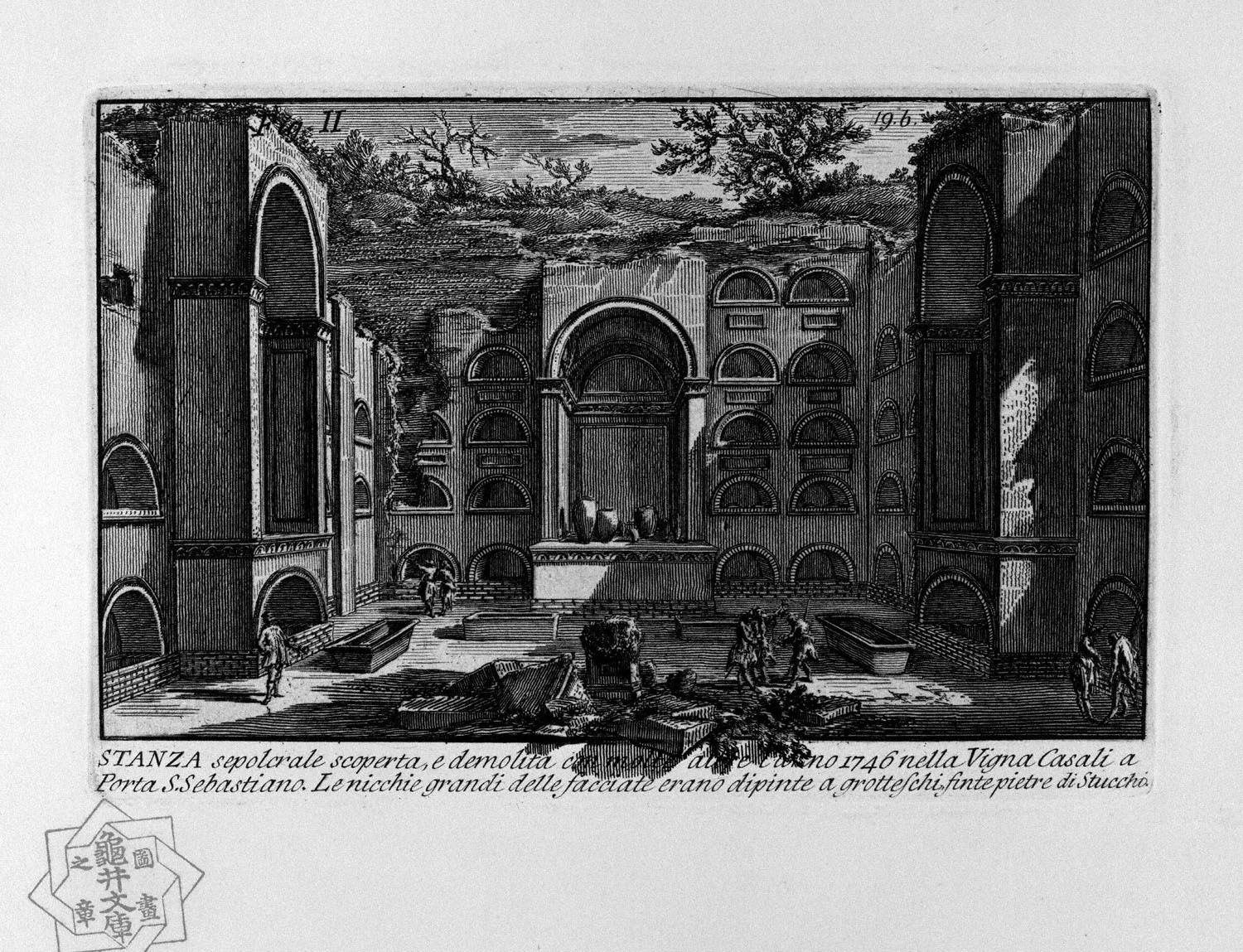This black and white charcoal drawing depicts the interior of an enormous, seemingly roofless building. The structure is characterized by its tall walls adorned with numerous archways and semicircular cutouts, some resembling shelves or cabinets. Despite its indoor impression, the absence of a ceiling reveals an exterior backdrop of grassy hills and trees sprouting from the top, creating an open-air effect. Central to the scene are troughs or bathtubs that hint at the space being used as a market or communal area. The scale of the building is emphasized by a diminutive figure in the bottom left corner. Detailed line work and vertical lines cover the scene, with some text—possibly including the word "stanza" and other unreadable lines—along the bottom edge. Additionally, a unique drawing resembling a Star of David with intricate writing appears in the lower section, all bordered by a light blue frame.